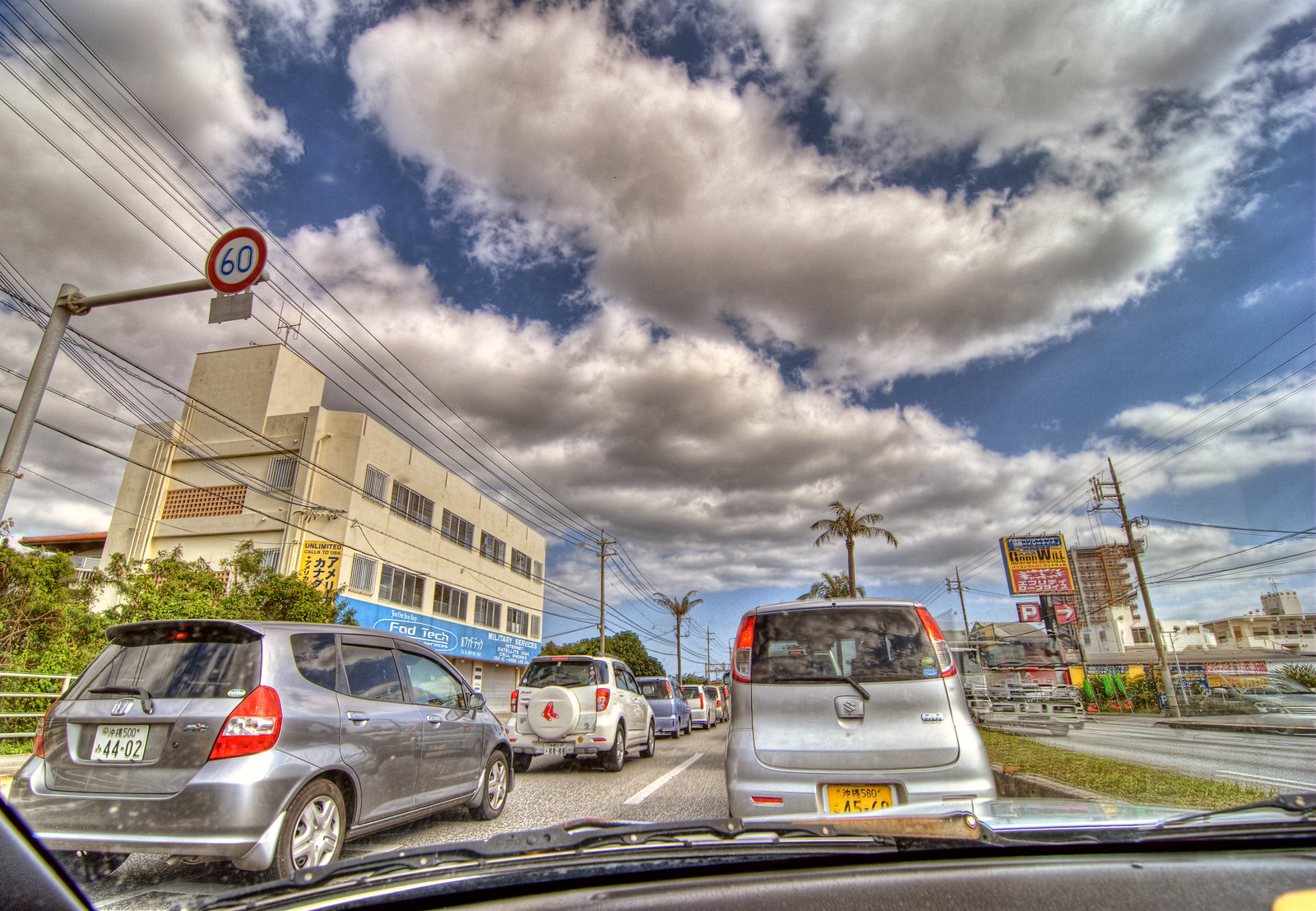The photograph captures a moment during a traffic stop or at a red light, showcasing a scene viewed from inside a car. The interior of the car is barely visible, with only parts of the black or gray dashboard and the windshield wipers in the foreground. Ahead, there is a gray car directly in front, a gray car to the left, and a white car further ahead. Multiple cars can be seen in the distance, indicating a busy roadway.

To the left of the image, a red circular speed limit sign with the number "60" prominently displayed stands near a cream-colored, two to three-story building adorned with several windows. Above, a clear blue sky is dotted with fluffy white clouds, adding a serene backdrop to the urban setting.

On the right side, several orange and red signs are visible, though their purpose is unclear. The scene appears to be a four-lane highway, as all visible cars are traveling in the same direction, separated by white dividing lines on the gray cement pavement.